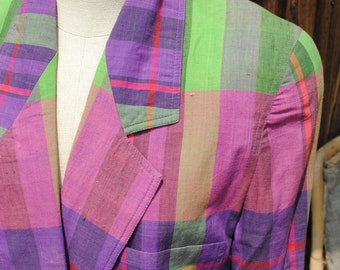This image features a white mannequin dressed in a plaid flannel shirt prominently displaying a variety of colors, including dark purple, magenta, dark green, light green, pink, and some thin red stripes. The shirt, which has the appearance of being thin, is wrapped around the mannequin's chest and has a large collar that adds to its distinctive pattern of horizontal and vertical rectangular shapes. The photo captures the mannequin from the chest upwards, showing only the left arm, shoulder, and part of the chest, while obscuring the head and legs. Notably, the right side of the mannequin is not visible. In the background, there is a chair positioned in the lower right corner with a gray back and a brown support, though it is partially obscured by the focus on the mannequin and the detailed plaid shirt it is wearing.